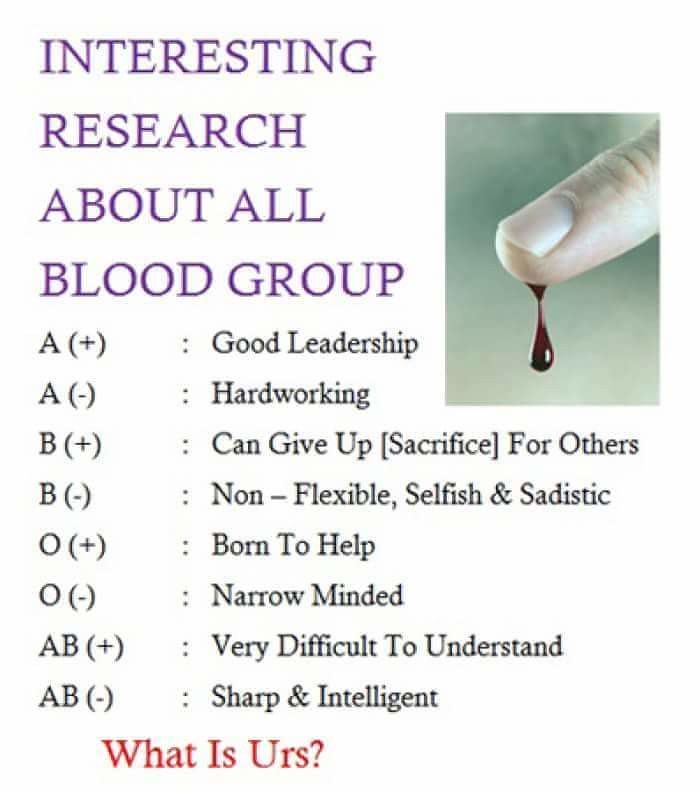This is a detailed poster titled "Interesting Research About All Blood Groups." Positioned on the right side of the title is an image of a white finger with a dark red drop of blood dripping from it, set against a green-black background. Below the title, a list categorizes personality traits by blood group:

- A+ (A positive): Good leadership
- A- (A negative): Hardworking
- B+ (B positive): Can give up (sacrifice for others)
- B- (B negative): Non-flexible, selfish, and sadistic
- O+ (O positive): Born to help
- O- (O negative): Narrow-minded
- AB+ (AB positive): Very difficult to understand
- AB- (AB negative): Sharp and intelligent

At the bottom of the poster, a bold question in red letters asks, "What is URS?" suggesting a call to the viewer's curiosity about their blood type and associated traits.